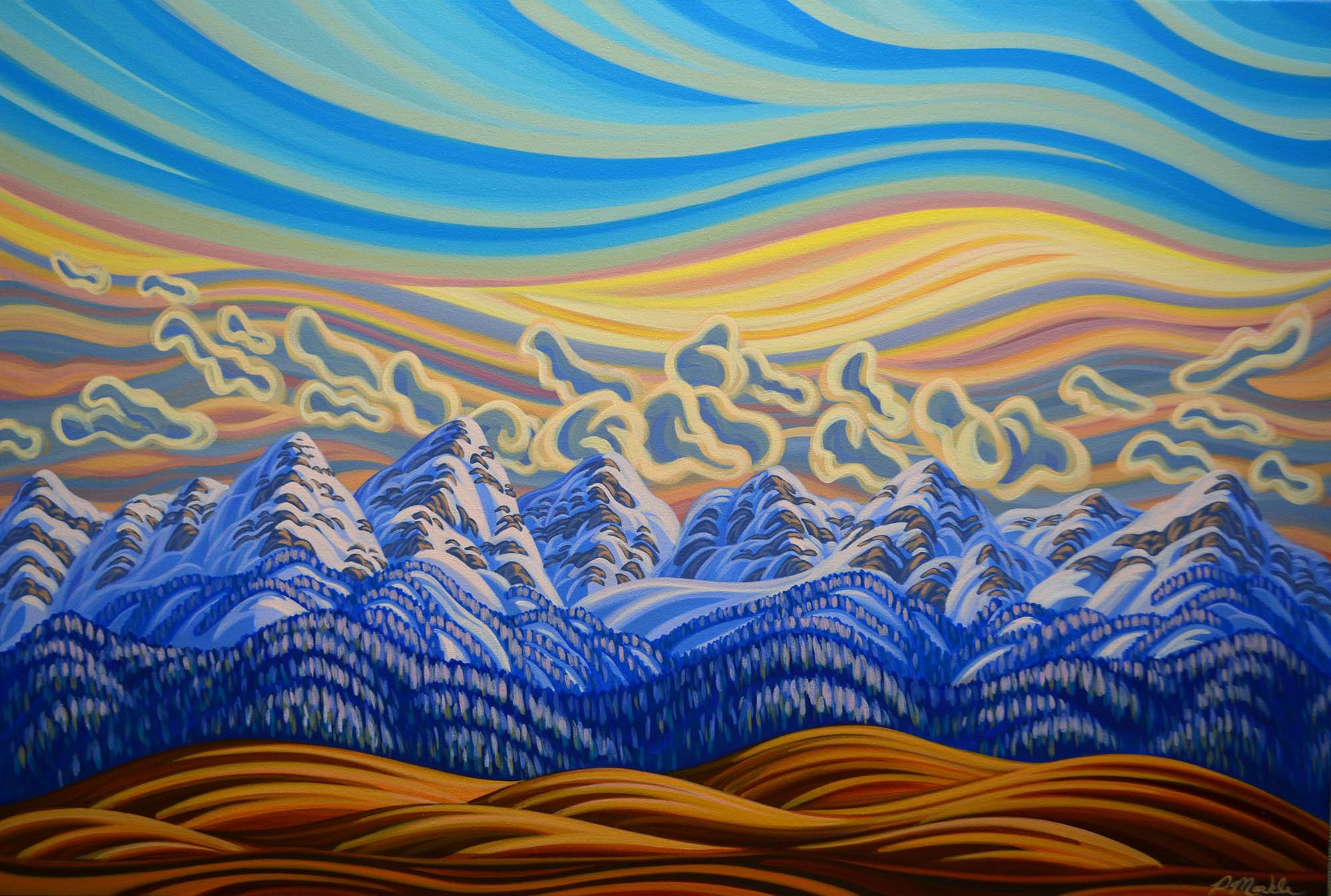This intriguing painting, potentially computer-generated, showcases a highly stylized and colorful landscape with multiple layers of vivid imagery. Starting from the bottom, the foreground features flowing brown waves resembling hills and valleys. Moving upward, these brown waves transition into blue waves with gray striations, implying dense clusters of trees. Just above this lies a range of prominent rocky mountain peaks, accentuated with white snow caps and a blue tint. In the midst of the painting, stylized clouds, blue at their core with light yellow outlines, add a dreamy quality. The background sky bursts with dynamic streaks and waves of vibrant colors, from yellow and orange to pink, blue, and reddish hues, creating a visually captivating and divided composition. Despite the diverse and abstract nature of the elements, the painting possesses no visible writing, people, animals, buildings, or motorized vehicles, encapsulating a raw, untamed natural scene.